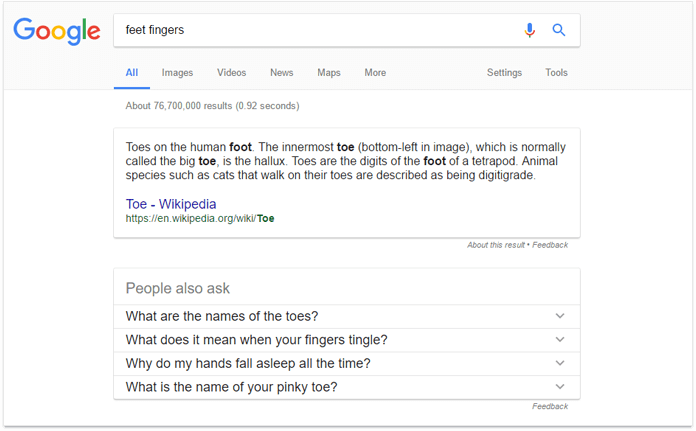The image captures a screenshot of a Google search results page. In the upper left-hand corner, the iconic multicolored Google logo is prominently displayed, featuring the letters in blue, red, gold, and green. The search query entered is "feet fingers," visible within the search bar which also contains a microphone icon and a search icon.

Directly beneath the search bar, navigation tabs are underlined in blue, indicating active and accessible options: "All," "Images," "Videos," "News," "Maps," "More," "Settings," and "Tools."

The first search result box provides detailed information about toes, stating: "Toes on the human foot. The innermost toe, bottom left in image, which is normally called the big toe, is the hallux. Toes are the digits of the foot of a tetrapod. Animal species such as cats that walk on their toes are described as being digitigrade." A link to a Wikipedia article on "Toe" appears in purple, preceded by a brief URL fragment "slash wiki slash toe."

Beneath this result, small print denotes options for "About this result" and "Feedback."

The subsequent result box labeled "People also ask" features commonly queried questions with associated drop-down arrows for further exploration: "What are the names of the toes?", "What does it mean when your fingers tingle?", "Why do my hands fall asleep all the time?", and "What is the name of your pinky toe?" Each question can be expanded for additional information. Below this segment, another "Feedback" option appears in small print.